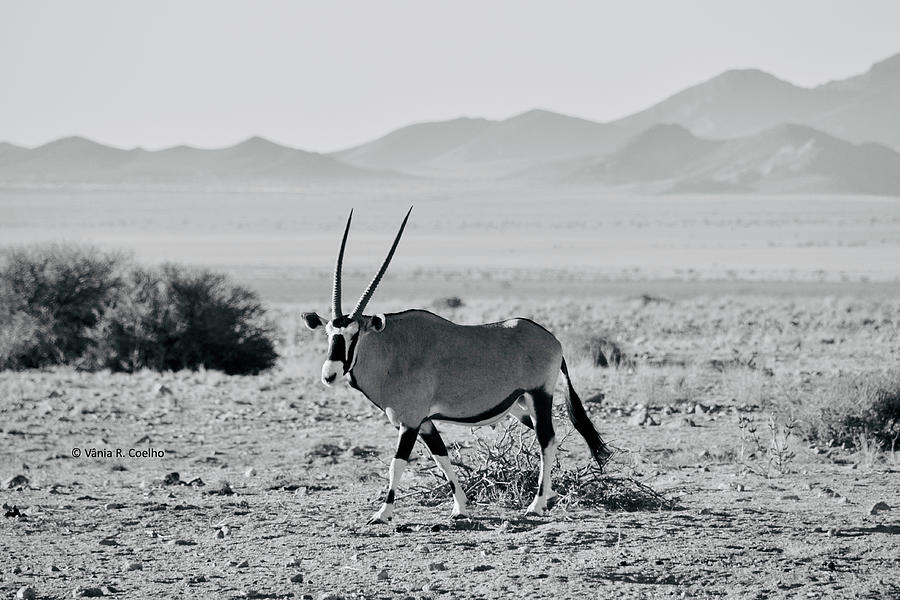This is a black-and-white photograph capturing a solitary antelope-like animal standing centrally in an arid, flat landscape. The photograph, rectangular in shape, features longer top and bottom sides compared to the left and right sides. The animal, likely an antelope or impala, boasts two long, dark-colored horns, and its head displays distinctive white spots around the nose and eyes, complemented by black stripes and spots on its face, legs, and tail. Its body is primarily a tannish hue with white legs accented by black markings.

The surrounding environment is sparse, characterized by scattered clumps of vegetation, small round bushes with tiny green leaves, and dead shrubs. In the mid-left section of the photo, you can spot two partially-grown bushes resembling tumbleweed. The far background reveals a series of gray mountains, devoid of vegetation or snow, shrouded slightly by fog, adding depth to the scene. Between the foreground and the distant mountains, the hint of a traditional dirt road stretches out, reinforcing the desolate nature of the setting devoid of any human activity.

An additional detail includes a hidden copyright inscription, "Bania R. Colhoe," discreetly placed within the upper-left portion amidst the dirt road. The varying shades of tans and grays, coupled with the detailed textures captured in the monochromatic palette, enhance the stark beauty of this untamed landscape.